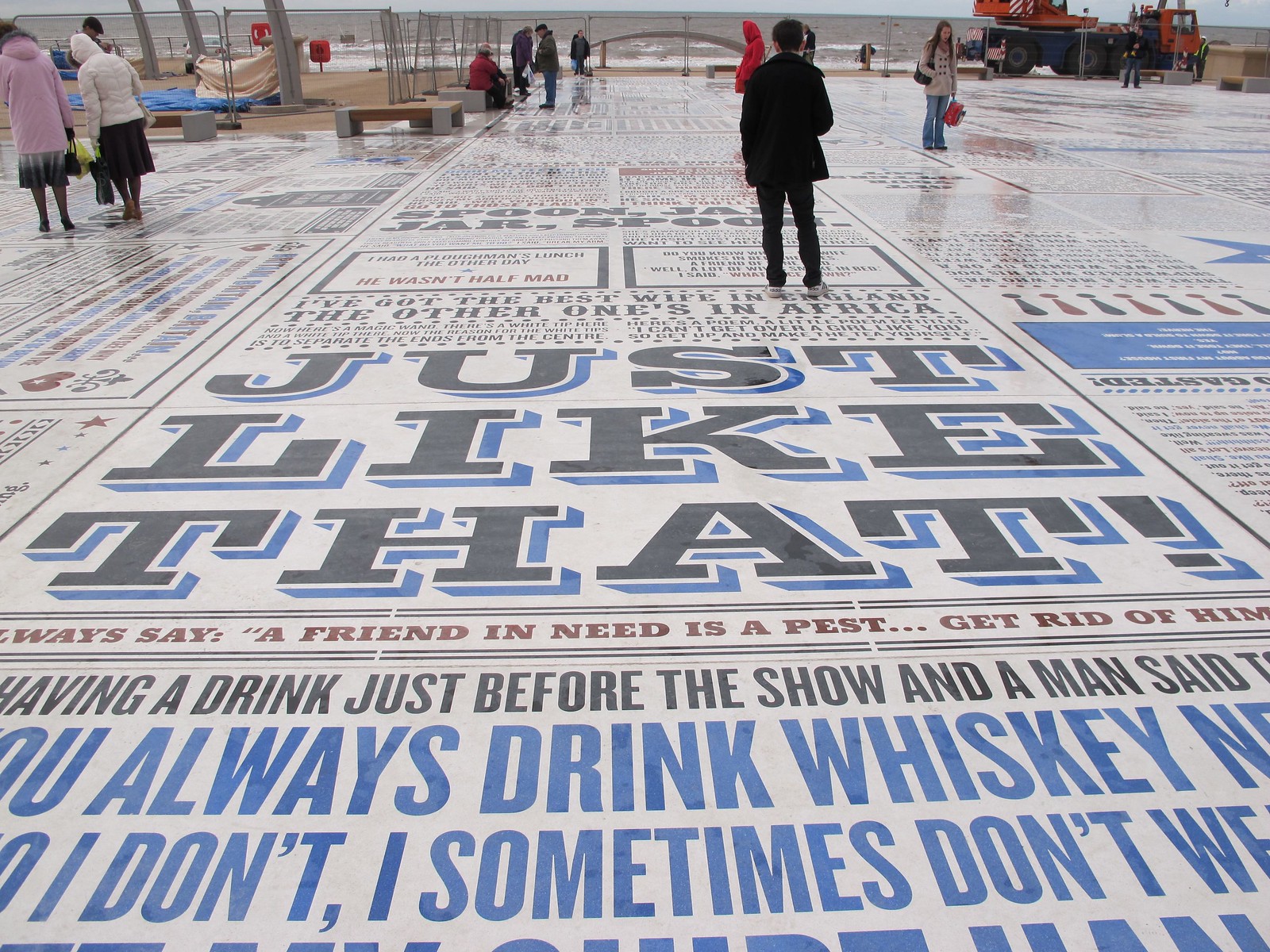This color photograph captures a unique scene at a beach. In the far background, the ocean and sandy shore stretch across the top of the image, under an overcast sky that suggests a cool, not sunny day. The main focus of the photo is a creatively designed walkway that dominates the foreground. This walkway, paved to resemble giant newspaper columns, features a striking combination of black, blue, and white elements, and is adorned with large, prominent lettering that states "just like that." Scattered throughout the walkway are various sentences, one of which reads, "you always say a friend in need is a pest, get rid of him."

Central to the image is a person dressed entirely in black, walking on this newspaper-print-like surface. Surrounding this individual, and further into the distance, are several other people. Most of them are wearing jackets or coats, indicative of the chilly day, and they seem to be examining the unusual text-covered walkway beneath their feet. Some benches and other objects can also be seen along the sandy portion of the beach in the background. This intriguing scene melds the artistic walkway with the natural beauty of the beach and ocean, creating a captivating and thought-provoking image.